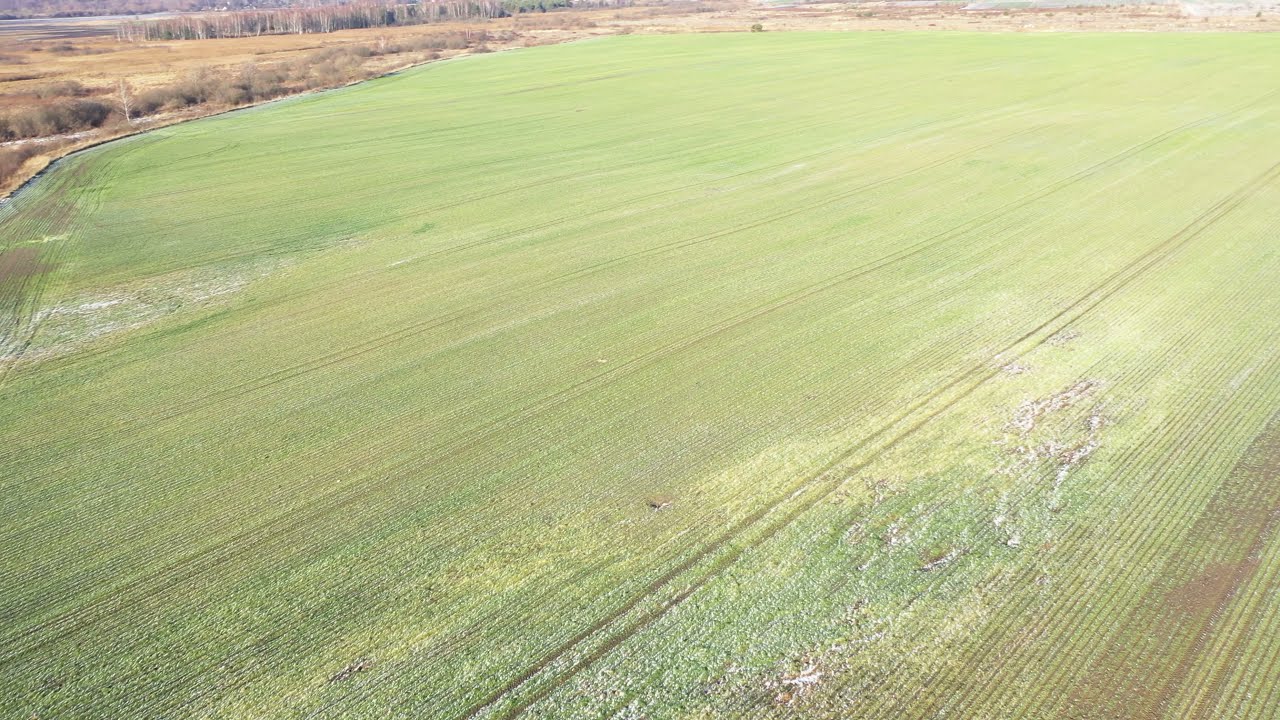This bright and sunny outdoor image, likely taken from a drone, captures a large expanse of farmland. The field is predominantly covered in light green vegetation with visible diagonal rows, suggesting it was recently cultivated or possibly harvested. Extending from the lower right to the upper left of the photograph, the field shows clear lines where crops were planted, interspersed with patches of dirt. Notably, tire tracks from farm equipment snake diagonally from the bottom center to the right side. Bordering the field, the terrain shifts into a more rugged, marsh-like area characterized by golden yellow and brown hues, with sparse, perhaps dying, trees, indicating a transition into late summer or early fall. The overall scene underscores a stark contrast between the cultivated green field and the wild, untamed surroundings.